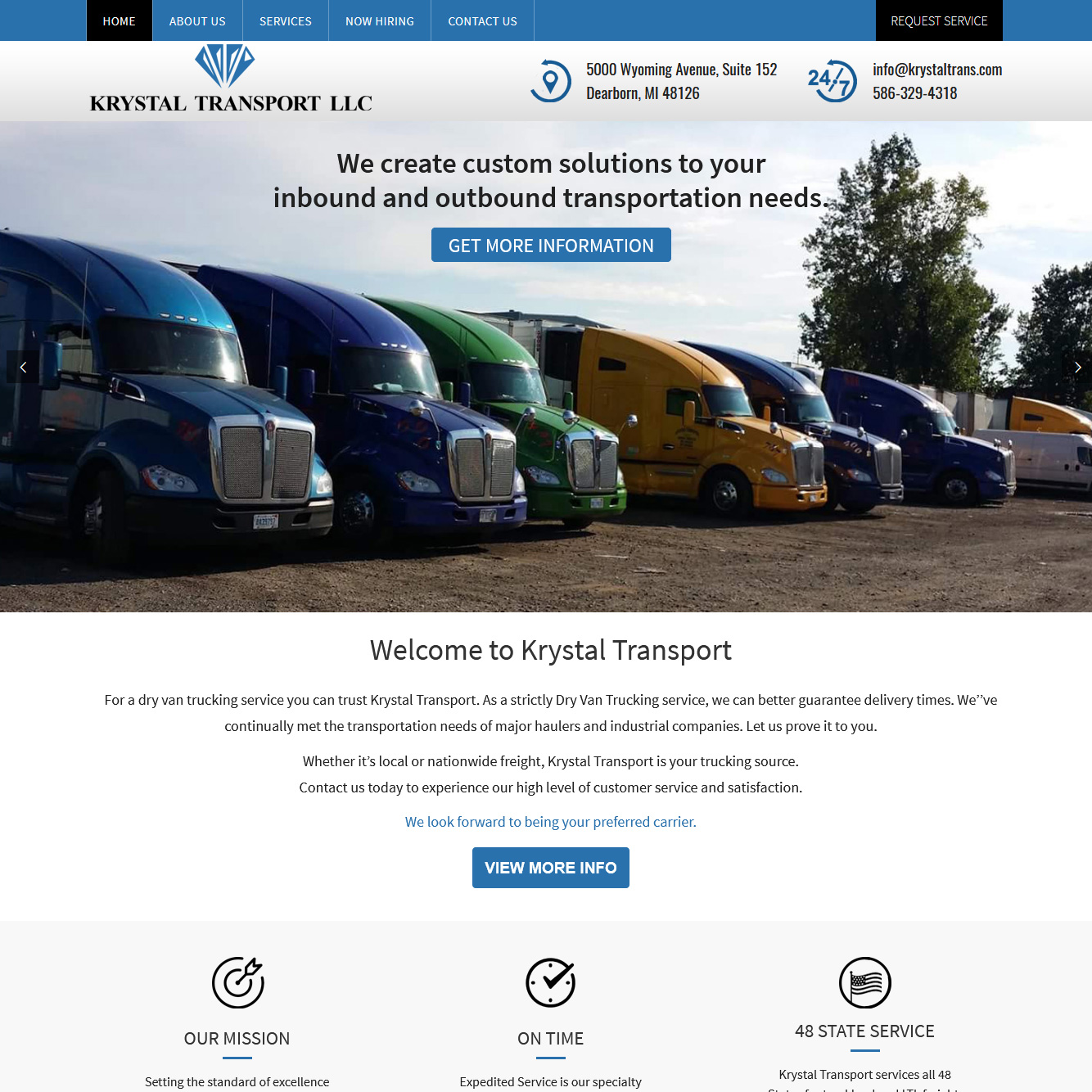Welcome to Crystal Transport

Located at 5000 Wyoming Avenue, Suite 152, Dearborn, MI 48126, Crystal Transport specializes in custom solutions for all your inbound and outbound transportation needs. We pride ourselves on being a reliable, strictly dry van trucking service, ensuring timely and efficient deliveries.

Our fleet consists of a variety of vehicles including a blue truck, a darker blue truck, a green truck, a yellow truck, a black truck, a purple truck, a white van, and multiple semi-trucks— all set against a backdrop of green trees and cloudy skies.

Since our inception, we've continually met the transportation needs of major haulers and industrial companies, proving our commitment to excellence. We offer services both locally and nationwide, always striving to be your preferred carrier.

For more information or to request our services, visit our website at krystaltrans.com or email us at info@krystaltrans.com. You can also reach us by phone at 586-329-4318. Let us demonstrate our high level of customer service and satisfaction. Crystal Transport is dedicated to setting the standard of excellence with on-time, expedited service. Contact us today and experience the best in dry van trucking.